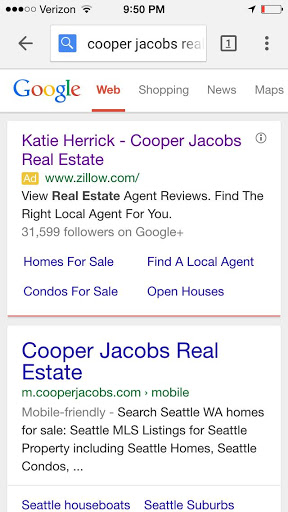This is a detailed screenshot of a mobile phone displaying a Google search for "Cooper Jacobs real estate." At the top, the phone's status bar is visible, indicating that the device is on the Verizon network with three out of five signal bars. Additionally, the Wi-Fi icon shows a strong signal, and the time is 9:50 p.m. Other status icons include a location arrow and a nearly depleted battery at roughly 20%, indicated by a red battery icon.

The Google search bar shows the query "Cooper Jacobs real estate." Below the query, the iconic Google logo is displayed in its blue, red, yellow, and blue-red colors. The search results are filtered by the "Web" tab, which is highlighted in red. Other available tabs include "Shopping," "News," and "Maps," displayed in gray.

The first search result is an advertisement marked with a small yellow "Ad" label, offering services from "Katie Herrick, Cooper Jacobs Real Estate" associated with Zillow.com. The ad includes options to find homes for sale, local agents, condos for sale, and open houses.

Below the ad, the primary search result is for Cooper Jacobs Real Estate, accessible via CooperJacobs.com. The site is noted to be mobile-friendly, allowing users to search for homes for sale in Washington state.